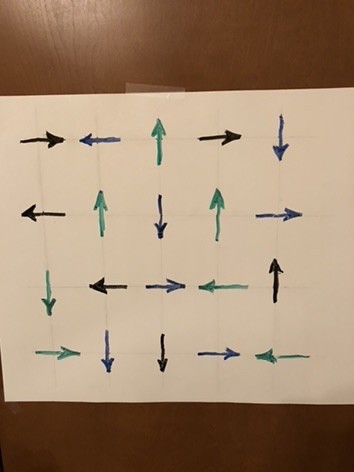The image features a white poster board taped against a dark brown background, either on a wall or lying on the floor. The poster board is adorned with hand-drawn arrows created using a magic marker or pen, forming an organized grid with five rows. Each arrow has a short, distinct stem and varies in direction and color.

- The first row contains two black arrows side by side, one pointing to the right and the other to the left.
- The second row consists of an arrow pointing left, an arrow pointing upward, another one to the left, and one pointing downward, all in various colors.
- The third row includes an arrow pointing up, one pointing down, another pointing right, and the last one pointing down again.
- The fourth row features four arrows: the first one pointing right, the second green one pointing down, the third one also green pointing left, and the fourth pointing right.
- The fifth and final row contains a downward-pointing arrow, one pointing right, another pointing up, and the last pointing left.

Overall, the poster board displays a systematic arrangement of arrows pointing in different directions and colors, adding a sense of dynamic movement to the image.